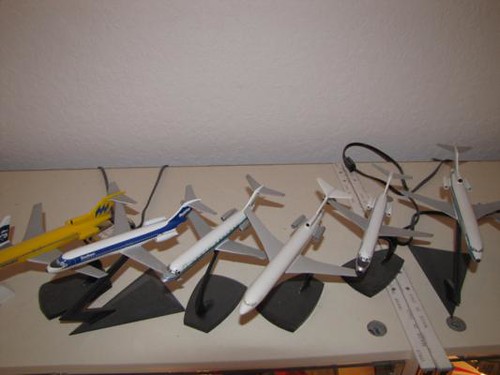This photograph captures a collection of six model airplanes meticulously arranged on a white shelf against a white wall. Each airplane is mounted on a black, four-sided platform. From left to right, the models include a predominantly yellow plane with gray wings, a white plane with blue stripes, and several predominantly white planes with silver or gray wings. The shelf seems to have a ruler or some straight object dividing it, adding a sense of structure to the layout. The planes, resembling jetliners, are all facing towards the camera. The white wall and shelf provide a clean backdrop, with a slight glimpse of a dark floor visible in the lower right corner of the image.